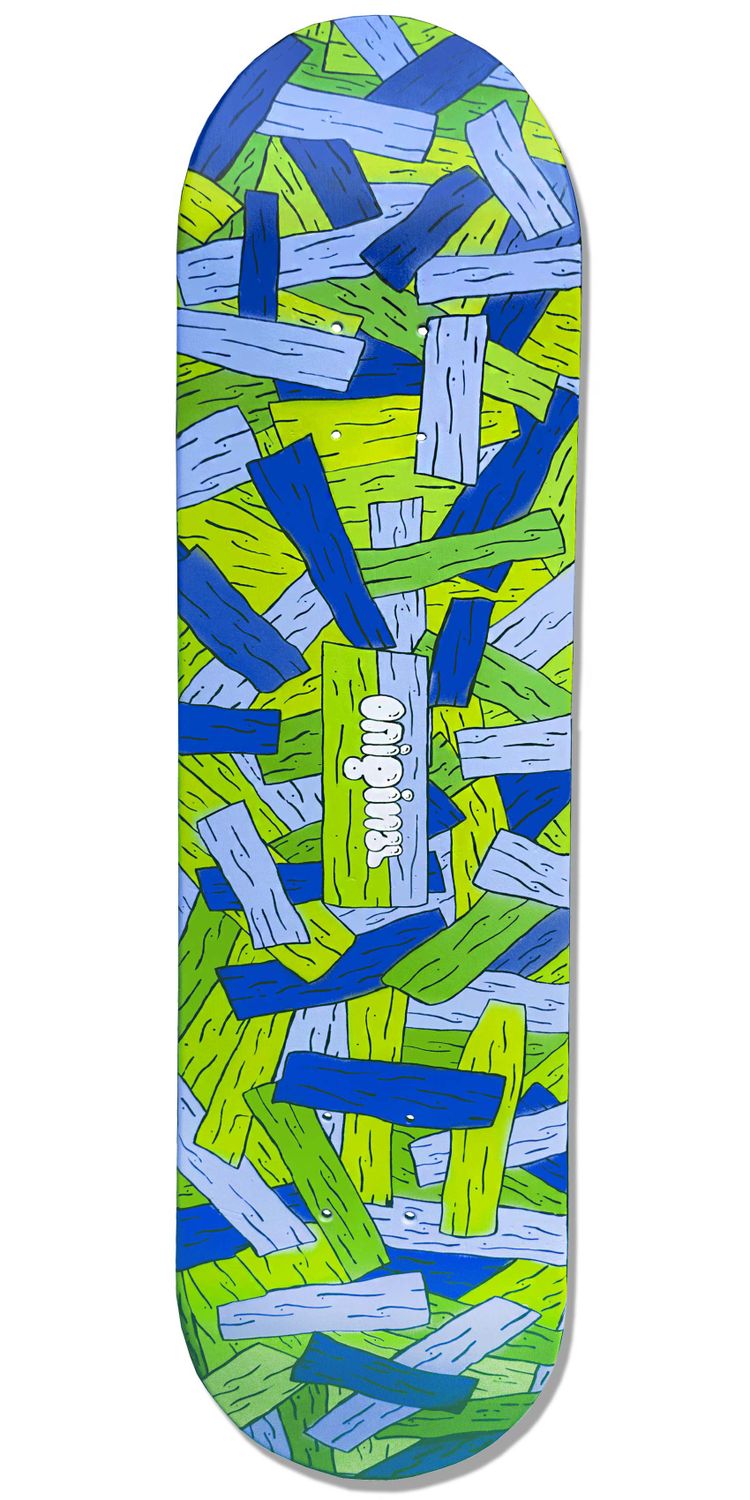This image depicts the bottom of a skateboard against a white backdrop. The skateboard has a distinct oblong shape with rounded ends. The surface is intricately adorned with a collage of irregularly shaped rectangles in shades of dark blue, light blue, and various greens. Each rectangle features black squiggly lines, arranged without any specific pattern, creating a visually dynamic design. Central to the skateboard is a rectangle that stands out, emblazoned with the word "Original" in prominent white bubble letters. The overall effect is a playful, cartoon-like aesthetic. Subtle shadows surround the skateboard, adding a touch of depth to the presentation.